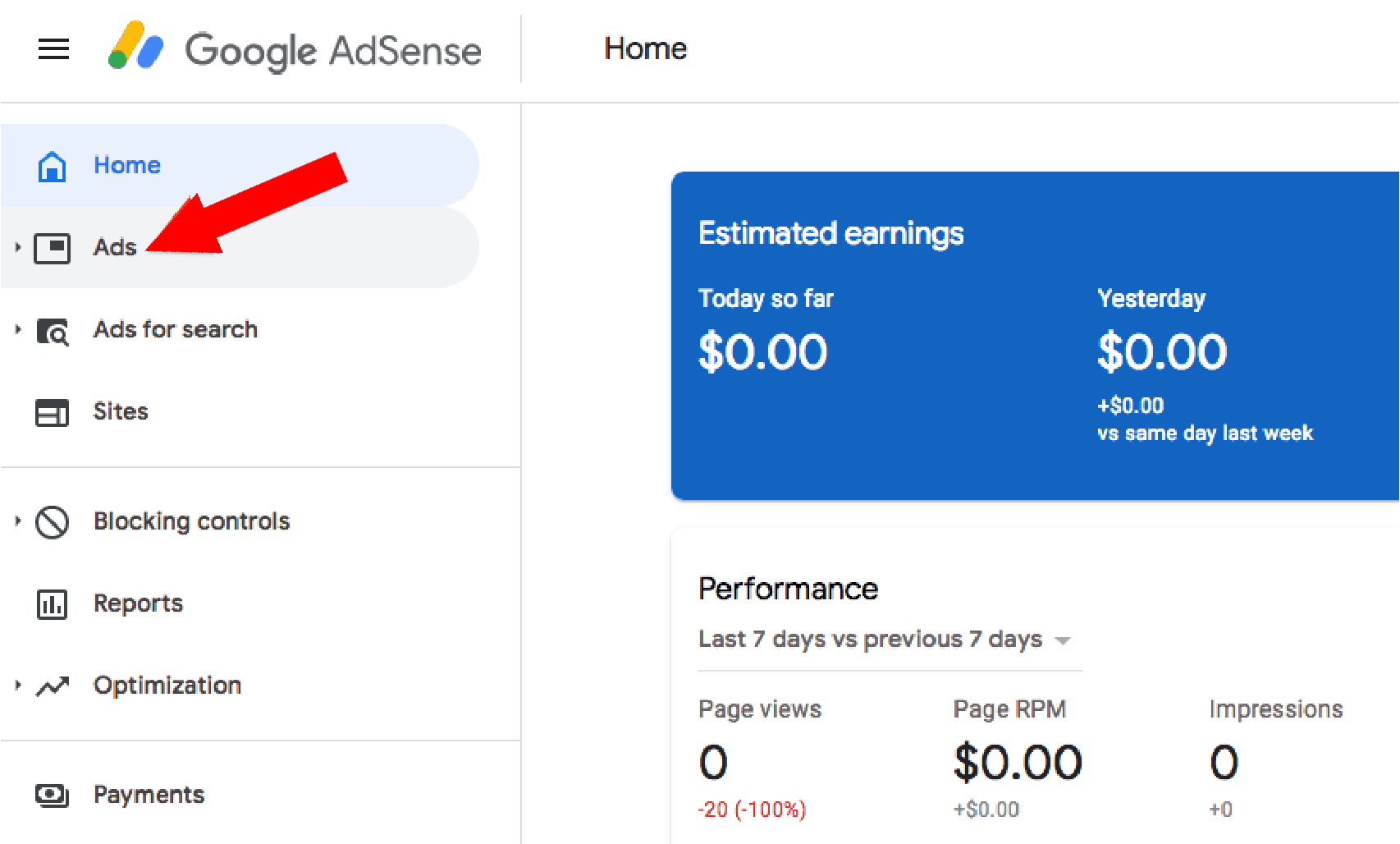A screenshot of the Google AdSense dashboard is displayed, showcasing various sections including Home, Ads, Ads for Search, Ads for Search Sites, Blocking Controls, Reports, Optimization, and Payments. The Home tab highlights the estimated earnings, notably showing $0 for both today and yesterday, and mentions zero earnings compared to the same day last week. Performance metrics over the last seven days are compared with the previous seven days, indicating 0 page views, a decrease of 20 views by 100%, and $0 in revenue per thousand impressions (RPM). Impression counts are also at zero, reflecting no change.